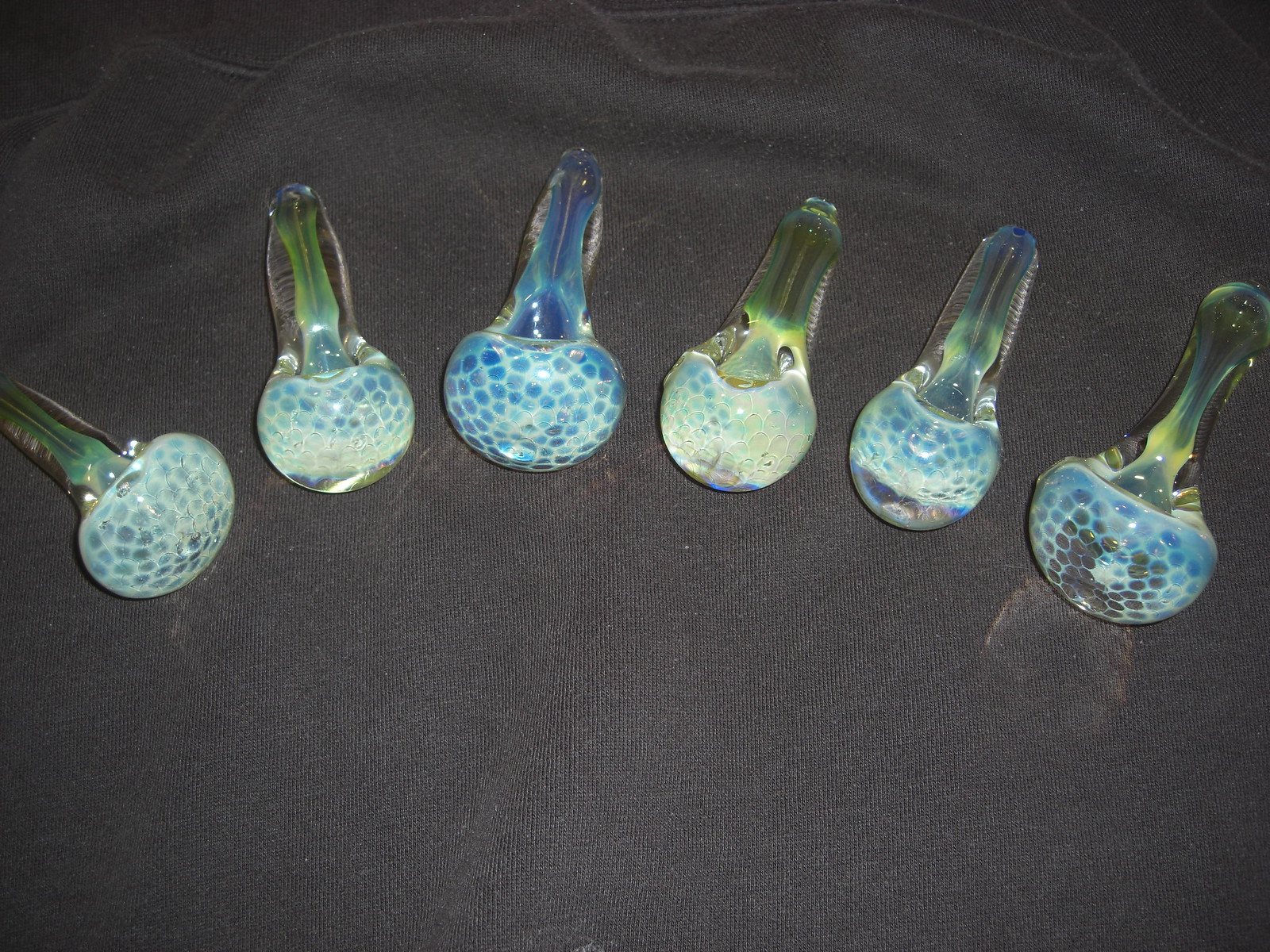This is an overhead picture of six custom-blown glass pipes, designed for smoking marijuana or tobacco. They feature a characteristically large, hollow bulb at the bottom, topped with a bowl for placing the substance. The pipes are arranged in a slight arc on a dark gray, almost black cloth. These handcrafted pieces showcase a blend of translucent colors, predominantly green, blue, and yellow.

From left to right:

1. The first pipe displays a green handle bordered with brown, culminating in a light blue bulb with dark blue, snake-skin-like patterns.
2. The second pipe mirrors the first but with its mouthpiece facing directly up.
3. The third, slightly larger pipe, presents a dark blue handle with brown touches and a dark blue bulb featuring light blue, scale-like patterns at its tip.
4. The fourth is identical to the first two pipes.
5. The fifth pipe resembles the larger third pipe but has a more slender body with a light blue handle bordered with brown and a light blue bulb adorned with dark blue, square-like skellings.
6. The sixth pipe has a handle that transitions from yellowish blue to light blue, ending in a dark blue bulb with slight brown skelling at the front. 

These intricately designed, see-through glass pipes highlight the artisanal craftsmanship involved in their creation.